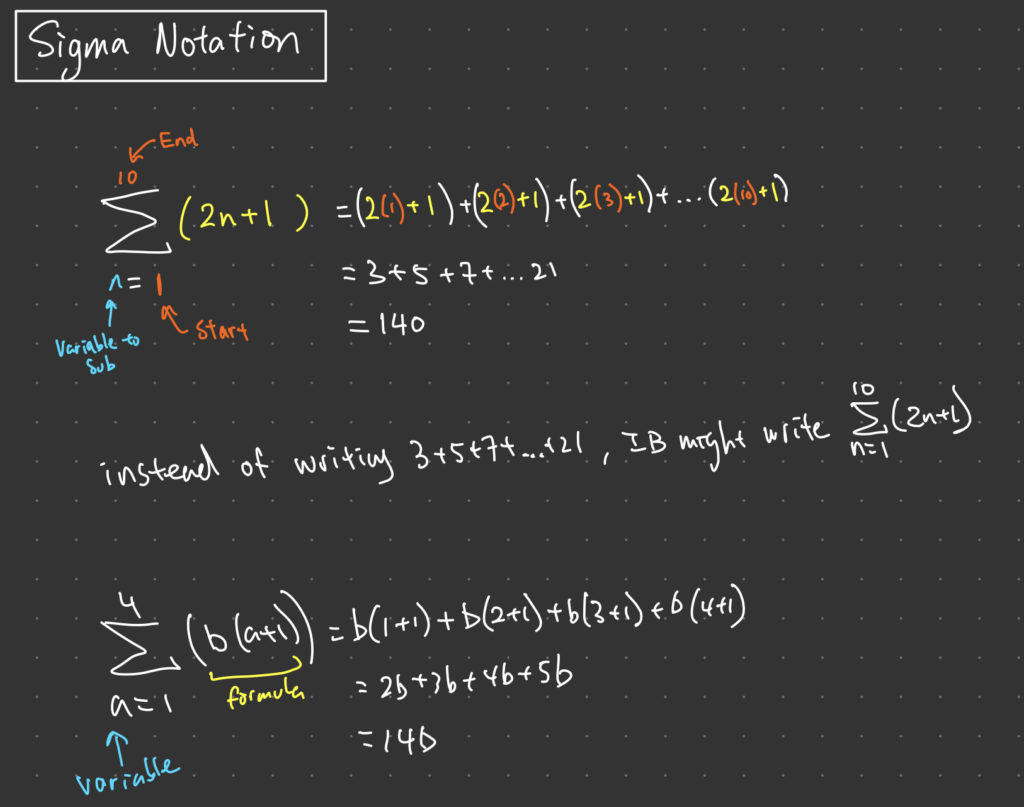This image displays advanced sigma notation mathematics, likely computer-generated but resembling handwritten text. The background is black with a grid of small white dashes, both horizontally and vertically aligned. In the upper left-hand corner, a white rectangular outline encloses the title "sigma notation." The main content consists of complex mathematical formulas primarily in white, with supplementary elements in red and yellow.

The formula is a demonstration of sigma notation, where the Greek letter sigma (Σ) is used to denote the summation of a series. The series is represented with subscript and superscript indicators, starting from 1 to 10. Arrows point to the sigma notation, illustrating its structure. The primary equation shown is "2n + 1," which expands into a sequence: "2(1) + 1," "2(2) + 1," continuing up to "2(10) + 1." This results in the terms 3, 5, 7, and so forth, summing to a final result of 140. Below this, an alternate method for expressing the same mathematical concept is provided, offering a different notation for clarity.

This detailed representation of sigma notation aims to provide a comprehensive understanding of the summation process, illustrating the intricate steps involved in advanced mathematical calculations.